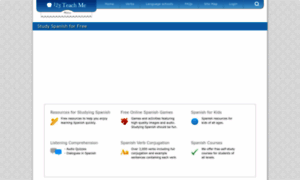The screenshot depicts a website interface, highly zoomed out to the point where the specific text is illegible. At the highest point of the visible screen, there is a navigation bar displaying a gradient from dark blue on the top left to a transparent light blue towards the center and right. Beneath the navigation bar, a white line is apparent, possibly designating the area for a drop-down menu associated with the dark blue section of the navigation bar.

Following this is a dark blue rectangular area that stretches horizontally off the edges of the visible screen, situated just below the white line. Below this, a vast expanse of white space is present, appearing somewhat empty and out of place compared to the rest of the page structure.

At the bottom portion of the screenshot, six clearly defined categories are arranged in a grid, with three categories per row. Each category is identified by a distinct icon:
- Top row, from left to right: a yellow icon, a red icon, and a dark blue icon.
- Bottom row, from left to right: a green icon, another yellow icon, and a gray icon.

However, the functionality or labels of these categories are not discernible due to the zoom level. The overall layout hints at a potential content section or dashboard interface, but the excess white space suggests incomplete content loading or an area reserved for dynamic content.